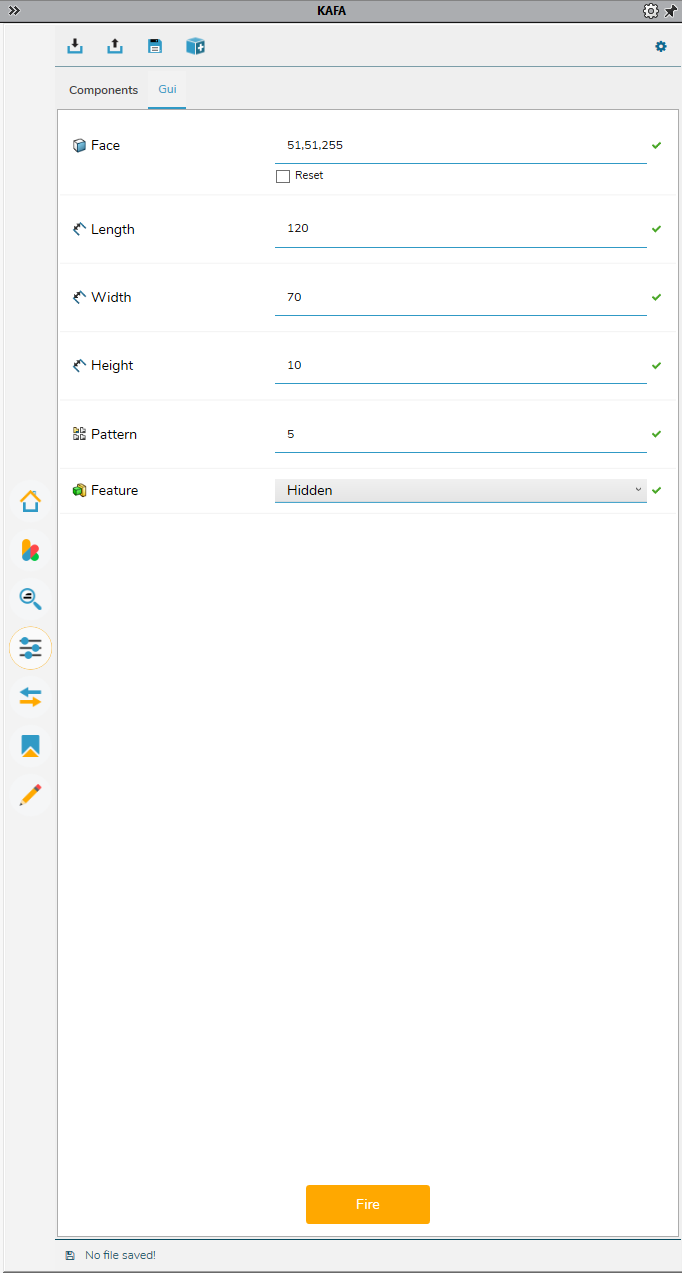The website interface features a top navigation bar with a gray background and the text "KAFA" prominently displayed in black at the center. To the left, there are two right-facing arrows, while the right side includes a settings icon and a thumbtack. Just below this bar, on the left, resides a row of icons in blue and black for download, upload, save, and an add new item function, followed by a thin blue line. 

Beneath this line, two tabs are visible: "Components" and "GUI". The "GUI" tab is currently selected, signified by its blue color and the blue underline beneath it, whereas the "Components" tab is black.

The main content area consists of a white background with a form-like interface. On the left, labels are listed sequentially with corresponding input fields and green check marks on the right. The form starts with "Face" alongside a value of "5151255" and a green check mark. Below this, the "Box" option is available with a footer saying "Reset" which is unchecked. Subsequent fields include "Length: 120", "Width: 70", and "Height: 10" each followed by green check marks.

Next, the "Pattern" field contains the value "Five" and features a green check mark. The "Feature" field has a dropdown menu displaying the option "Hidden" on a gray background with the text in black, also accompanied by a green check mark. All these options are separated by teal blue lines.

At the interface's bottom, a prominent yellow button labeled "Fire" is positioned.